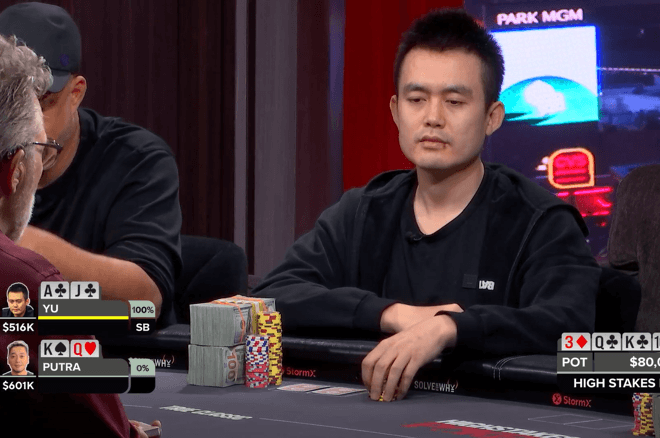The screenshot captures a riveting moment from a high-stakes poker game at Park MGM. The focal point is on a player named Yu, who has a serious and focused demeanor, exemplifying the quintessential poker face. He is of Asian descent, sporting black hair and a black sweatshirt. In front of him, prominently displayed, are two large bundles of $100 bills, amounting to approximately $20,000, and an array of poker chips. Yu's hands are poised over a stack of chips, indicating his intention to make a move. The pot stands at a staggering $80,000, emphasizing the high-risk nature of the game. Additionally, the screen shows another player named Putra, who is currently Yu's opponent in this tense hand. Both players' winnings are tallied—Yu with $516,000 and Putra with $601,000. The lower right corner of the image highlights the text "high stakes," reinforcing the intense atmosphere. An infographic on the left side details the current hands and winning odds of the players. The image immerses you into an eye-level view, as if seated at the table, caught in the intense atmosphere of professional poker.